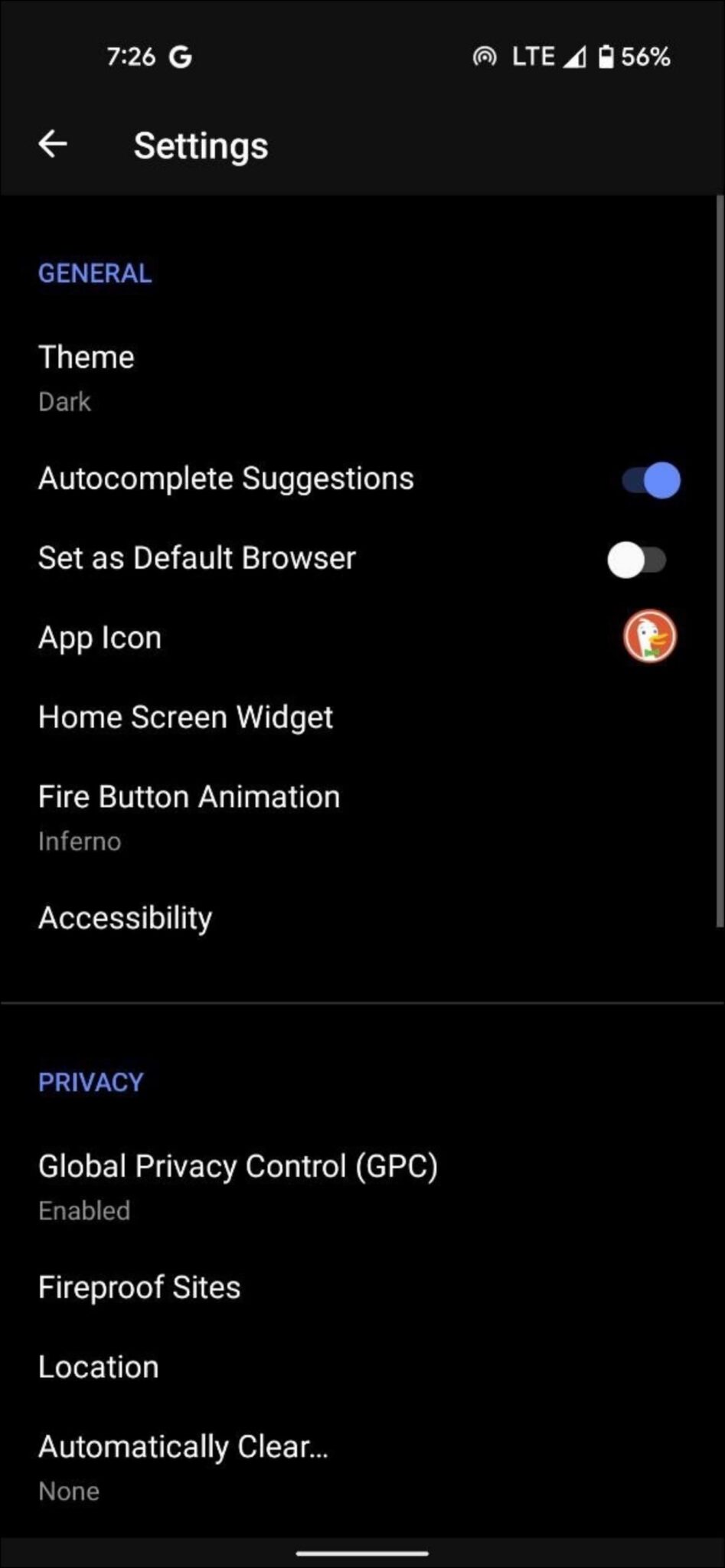A detailed view of the settings in the DuckDuckGo mobile app on Android is displayed. The interface is set to a dark theme, with an option to switch back to light mode if preferred. The app's logo is clearly visible in the section labeled "App Icon," confirming the browser's identity. Autocomplete suggestions feature is activated, while the "Set as Default Browser" option remains off. Users have the ability to choose a home screen widget from the available selections. The Fire Button animation is configured to the "Inferno" mode. The settings menu includes an accessibility subsection and a comprehensive privacy area. Within the privacy settings, Global Privacy Control is enabled, and the option for managing Fireproof sites requires further interaction. Location settings show an option for automatic clearance, reflecting various customization capabilities within the DuckDuckGo browser settings on the Android platform.